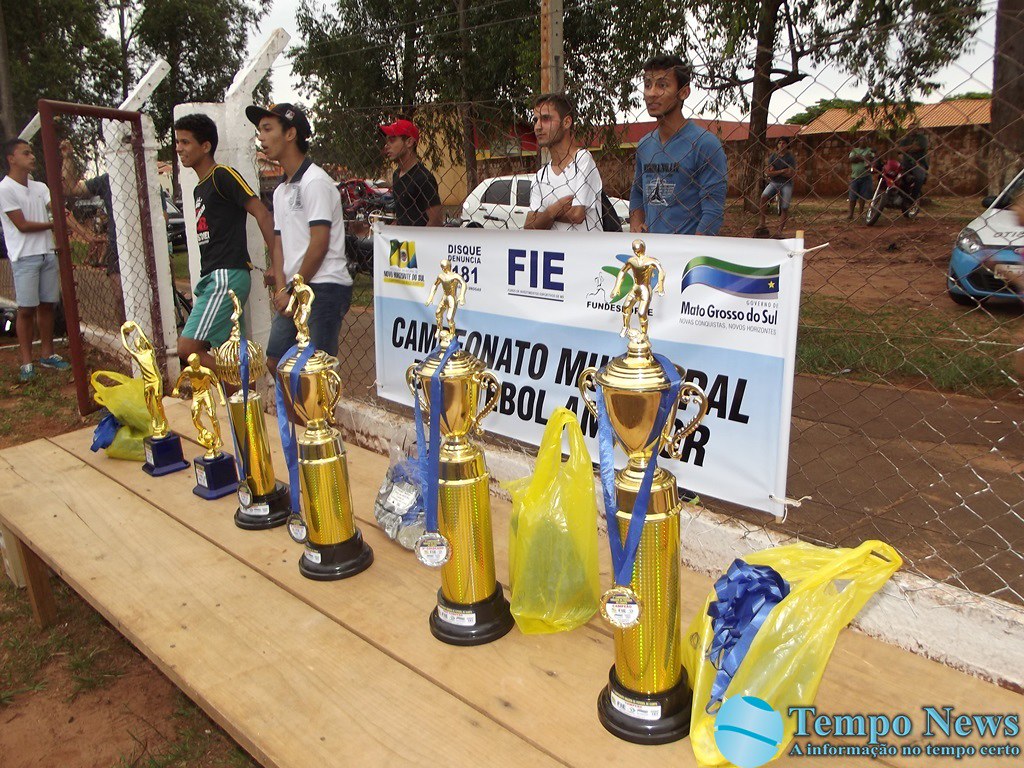The photograph showcases six progressively larger gold trophies displayed on a wooden bench outside near a field, possibly a European football field. In the background, a chain-link fence can be seen, with a banner attached that reads "Disk 181" on one side and "Mato Grosso do Sul" on the other, suggesting a location in Brazil. The trophies, presumed to be for soccer, feature golden muscular male figures on top, complemented by blue ribbons and gold-white emblems. Behind the fence, six gentlemen are watching the game intently, while three people are near a motorcycle in the distant background. The photo is marked with a caption in the bottom right corner: "Tempo News, Informativo no Tempo Certo."